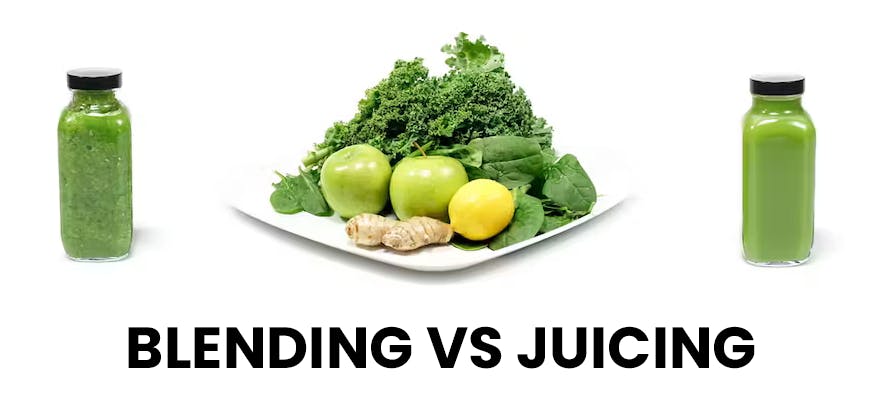The clean, horizontally rectangular, full-color photograph, likely staged and digitally enhanced, features a stark white background. Prominently displayed at the bottom in bold, capital black letters is the text "BLENDING VERSUS JUICING." At the center of the image, there's a square white plate laden with a variety of fruits and vegetables including green apples, a lemon, kale, spinach, and what appears to be brown ginger root. Flanking the plate are two similar clear glass bottles with black lids. The bottle on the right contains a smooth green liquid, while the one on the left holds a chunkier green mixture with apparent sediment. Subtle shadows beneath the plate and bottles add depth to the otherwise minimalistic composition.